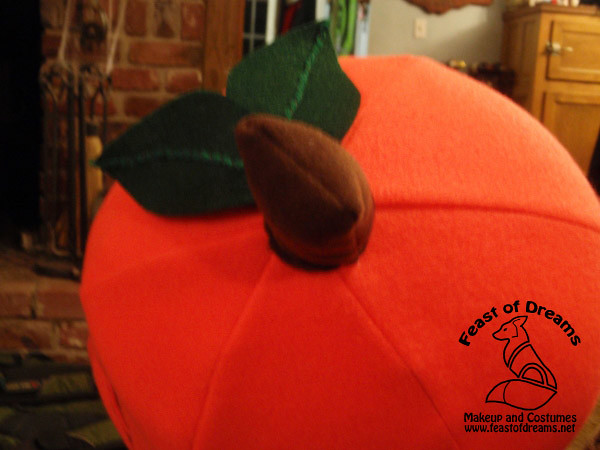This slightly out-of-focus, full-color indoor photograph prominently features a large felt pumpkin lying on its side, showcasing its orange surface, green leaves, and brown stem. Situated in the lower right corner is the company logo and name, "Feast of Dreams," with a fox illustration above the words "Makeup and Costumes" and the URL "www.feastofdreams.net." The background comprises a red brick fireplace equipped with metal pokers and stokers, a lightly stained tan oak dresser, and a white or off-white window. The setting is completed by a throw rug placed in front of the fireplace.